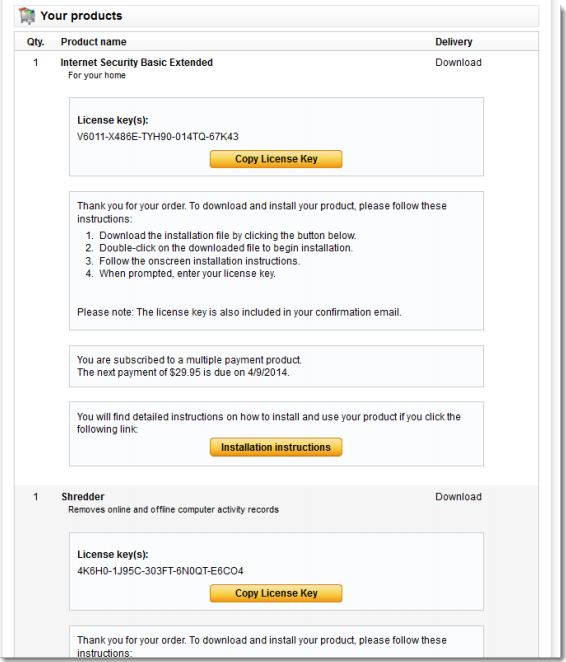The web page displays a detailed receipt for purchased digital products, starting with the header "Your Products." The first section lists the quantity, product name, and delivery type. 

- **Product 1**: Internet Security Basic Extended
  - **Quantity**: 1
  - **Delivery**: Download
  - **License Key**: Provided with a copy button
  - **Instructions**: 
    1. Download the installation file using the specified button.
    2. Double-click the downloaded file to start installation.
    3. Follow the on-screen instructions.
    4. Enter the license key when prompted.
  - **Additional Information**: The license key is also included in the confirmation email. 

A note specifies that the customer is subscribed to a multi-payment plan, with the next payment of $29.95 due on April 9, 2014. Another box offers a link to detailed installation and usage instructions via an orange "Installation Instructions" button.

- **Product 2**: Shredder
  - **Quantity**: 1
  - **Description**: Removes online and offline computer activity records.
  - **Delivery**: Download
  - **License Key**: Provided with a copy button

Each product section is accompanied by clear, step-by-step instructions for download and installation, ensuring the user can easily access and set up their newly purchased software.